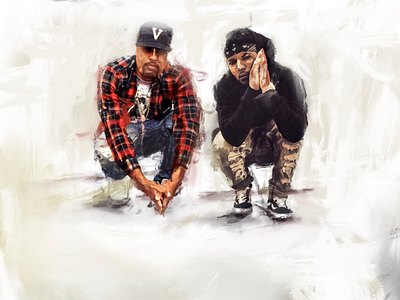The image appears to be an illustration set against a predominantly white background, accented with light beige paint strokes. It features two men, both crouched down next to each other. The man on the left is possibly of Latino descent. He sports a black baseball cap with a white "V" emblem, a red and black plaid long-sleeved shirt layered over a white graphic t-shirt, blue jeans, and white sneakers. His hands are clasped together in front of him. The man to his right also appears to be Latino, wearing a black bandana and a black hoodie with the hood partially up. He dons ripped jeans and black Vans with white soles. His hands are positioned in a gesture that could be interpreted as praying or resting, placed next to his face. Both figures seem to be in a contemplative or reflective pose, adding depth to the artist's depiction.